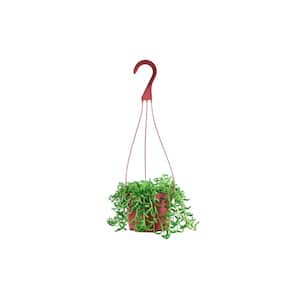This color photograph, presented in a square format on a completely white background, features a small red plastic hanging basket. The basket is suspended by three strands that converge at the top to form an orange hook. This hook and the strands extend above the basket, while the foreground of the image showcases a lush green plant with long, leafy stems. The stems cascade over the edges of the basket, trailing down to just graze the ground. Despite being a small, somewhat thumbnail-sized image, the photograph captures the intricate details of the plant's vibrant foliage and the basket's distinct strands and hook, which are notable in profile against the minimalist backdrop.